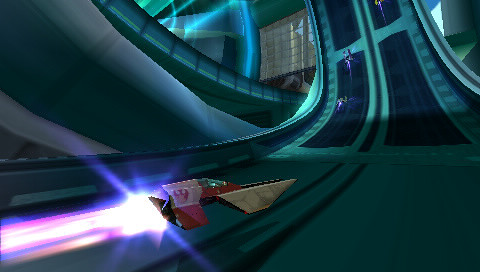This still image, taken from a video game, showcases a small, red and light gray spaceship with a see-through, bluish-tinted cockpit. The spaceship is racing up a green, neon-illuminated track that starts horizontally and curves steeply upwards into a vertical climb. Behind the spaceship, a vibrant trail of pink, purple, and white light bursts out, forming a starburst that accentuates its high-speed takeoff. The track itself is complex, featuring sections that are transparent and some made of reflective metal, giving it a futuristic, somewhat difficult-to-decipher appearance. The track appears to be segregated into two lanes with guardrails, and there are other similar-looking vehicles in front, emphasizing the competitive race environment.